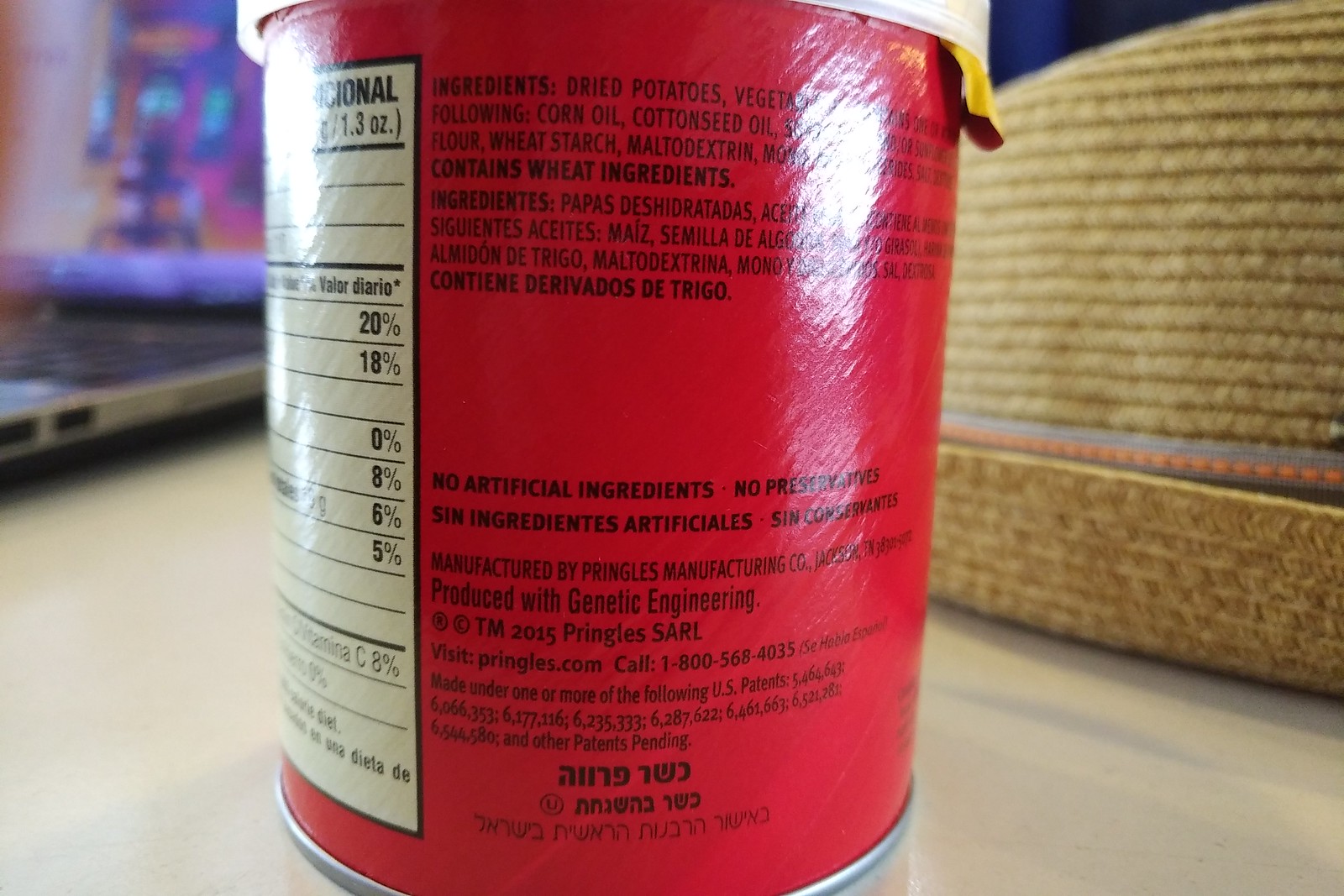This detailed, realistic photograph depicts a close-up view of a red Pringles can, which is prominently displayed in the center of the image with its ingredient list visible. The can, made of cardboard or paper and capped with a white plastic lid, highlights ingredients such as dried potatoes and vegetables. Notably, there is Hebrew writing alongside the English text, suggesting bilingual labeling. The backdrop is blurred but reveals a mix of elements. On the left, an open laptop displays fuzzy red and orange designs, with a black keyboard partially visible. To the right, a wicker or straw item, possibly a hat with a distinctive stripe, rests on the surface. The base of the image features a light tan, hardwood-like texture, possibly a tabletop or floor. The photograph, featuring notable trademarks dated 2015, combines everyday objects into a textured and layered composition.